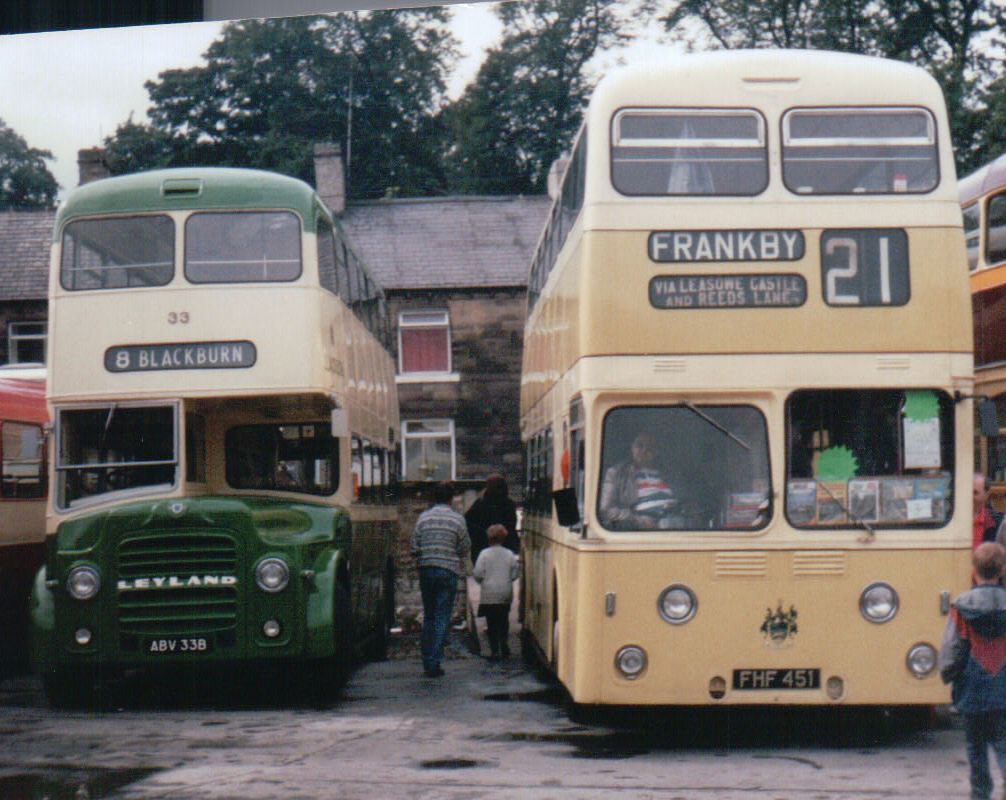This vintage photograph, characterized by its low resolution and faded colors, captures a nostalgic street scene featuring two double-decker buses facing the viewer. To the left, a green bus with a light tan body, labeled "8 Blackburn" and featuring the identifiers "Leyland" and "ABV33B," stands slightly smaller than its counterpart. Its cream and beige layers create a classic yet worn aesthetic. To the right, a larger, yellowish double-decker bus displays "Frank B 21," with routes "via Leesom," "Rees Lane," and the plate "FHF451." The driver is visible inside, seemingly awaiting passengers. In the gap between the buses, a mother and child walk towards the back, rendered almost as silhouettes against the bus's backdrop. The scene further includes a small boy standing near the front of the right bus. Brick buildings loom in the background, suggesting old residential structures, while the three-story building on the left features a chimney and a deteriorated roof. A blue sky dotted with leaves from tall green trees stretches across the top, further anchoring the image in a bygone era. To the far right, just above the boy's head, parts of another double-decker bus are partially obscured, adding depth to this historical streetscape.